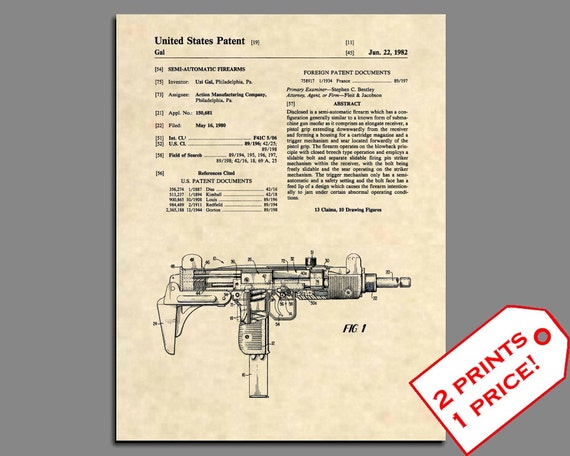Against a gray background lies an aged, yellowed piece of paper with the bold header "United States Patent" displayed in black. On the left, the term "gallon" appears, while on the right, the date "Jan 22, 1982" is marked. The document, which describes in detail the workings of a semi-automatic firearm, includes a detailed table of contents concerning the patent. Below, an intricate black and white illustration labeled "Figure 1" shows a semi-automatic firearm with its barrel pointing to the right, meticulously depicting its internal mechanisms such as pins, hinges, and the firing mechanism. In the bottom right corner of the image, a white tag with a red outline reads, "Two prints, one price," possibly indicating a sales promotion.